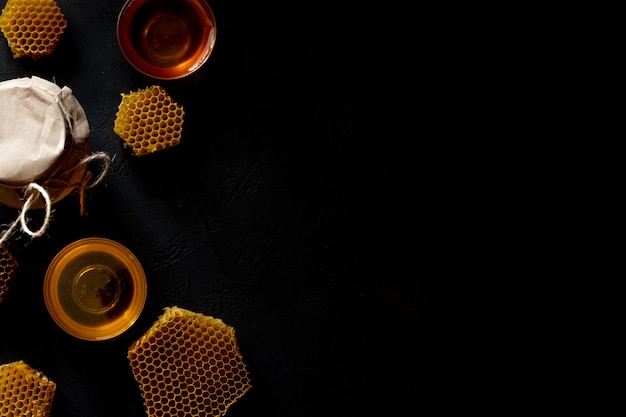The image is a top-down view featuring several objects associated with honey, all set against a fully black background, which covers three-quarters of the picture. On the left side, there are four golden honeycomb pieces, their hexagonal shapes displaying a glistening reflection of light. Interspersed among the honeycombs, there are two small circular dishes filled with honey. In the upper left corner, a small glass jar with a white paper covering secured by a string can be seen. This simple yet artistic arrangement showcases the honey and honeycomb theme, with the black background providing a striking contrast and possibly serving as a minimalist backdrop for creative or commercial purposes.